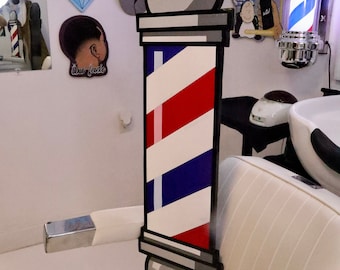The image depicts a well-lit barbershop interior with predominately white walls. Central to the scene is a white, padded barber's chair, complete with cushioned armrests reinforced with metallic ends. Positioned behind the chair is a white basin with a pronounced black neck rest, suggesting a shampooing station. Surrounding these main elements are various pieces of décor and accessories. A distinctive barber's pole—emblazoned with the traditional blue, white, and red stripes—appears twice: once as a lit, cylindrical object on the top right of the image, and again as a flat, cartoony illustration with black outlines on the chair. The back wall features artwork, including an illustration of the back of a Black man's head with a fade haircut, a New York sign, and a picture of Charlie Brown. Additionally, there is a mirror in the upper left corner reflecting parts of the barbershop. The overall ambiance of the space is bright and inviting, accentuated by ample lighting.